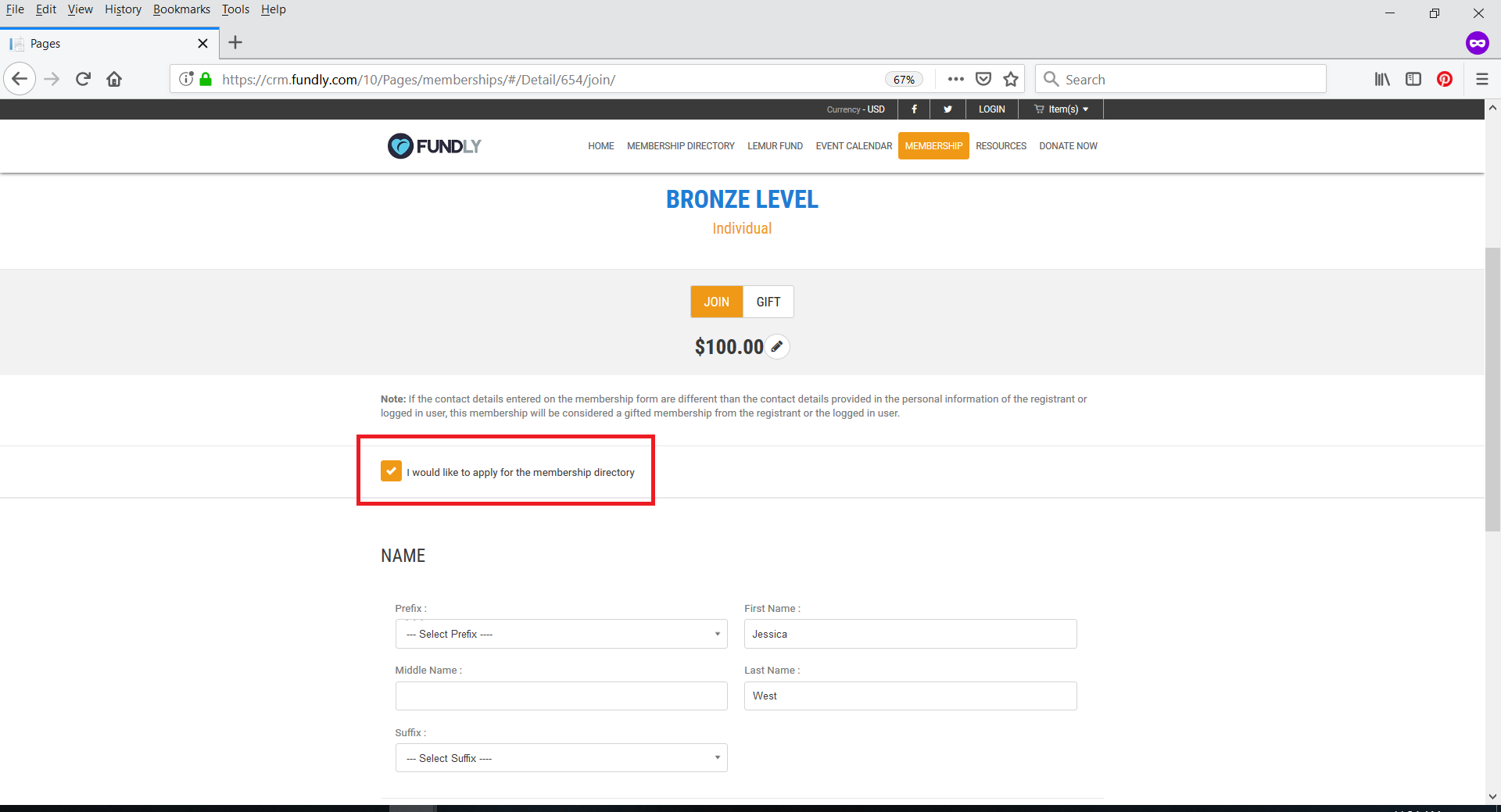Screenshot of a user interface displaying a web page on Fundly.com, specifically a membership sign-up page. The browser window shows common navigation elements such as File, Edit, View, History, Bookmarks, Tools, and Help. The address bar is secure, indicated by a padlock, and shows the URL: "https://cm.fundly.com/10/pages/memberships/details/654/join". The webpage features several interactive elements including a back arrow, forward arrow, refresh button, home icon, and more.

At the top menu, items like Home, Membership Directory, Lemur Fund, Event Calendar, Membership, Resources, and Donate Now are visible. 'Resources' has a gray highlight, and 'Membership' has an orange square highlight. The page displays different membership levels such as Bronze Level in blue and Individual in orange. There's a 'Join' button in white with an orange background, and a 'Gift Membership' option in black with a white background priced at $100.

An editable form section shows fields for Name, Prefix, Middle Name, Suffix, First Name, and Last Name, filled with an example name, Jessica West. There's a note indicating that if contact details on the membership form differ from those provided, the membership will be considered a gifted membership from the registered user. Additional elements include a red square highlighting an option to apply for the Membership Directory and selectable suffix options. This comprehensive user interface provides a detailed and visually structured approach to joining and managing memberships on the platform.